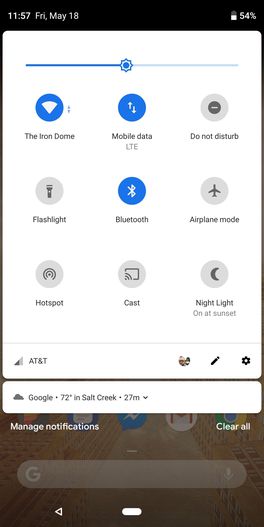A detailed view of a smartphone screen displaying various app icons and settings. The bottom section features a gray circle indicating the hotspot function, alongside icons for casting and a nightlight setting that activates at sunset. The display also shows an AT&T network, an edit button, and a settings icon. The weather information is prominently displayed, with "72°F in Salt Creek" and "27M" visible. Additionally, there are options to manage notifications, perform a Google search, and navigate back with a back arrow. In the background, a natural dirt trail is faintly visible, adding a touch of scenic beauty to the otherwise tech-focused image.